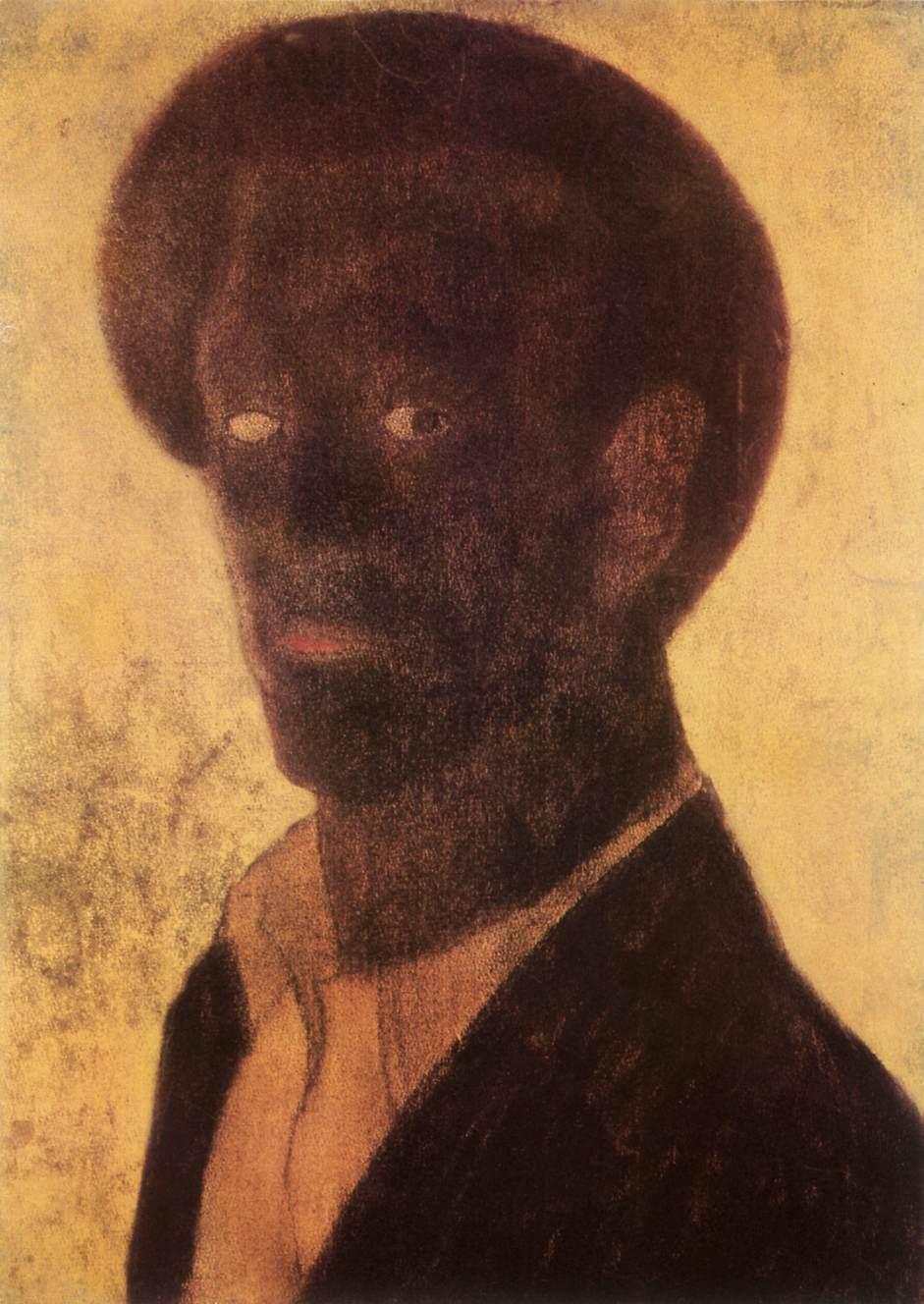The image is a detailed painting of a man, most likely an African American, set against a dirty yellow canvas background. His skin is very dark, creating a stark contrast with the light and yellowish hues behind him. The man is wearing a white button-down shirt with an open collar, beneath a dark, perhaps black, overcoat. His head is turned to face the viewer, though his body is angled away, adding a sense of dynamic tension to his pose. His left ear is prominently visible, large and distinct. His eyes are striking; the left eye shows a black pupil, while the right eye starkly displays only the white, giving an almost eerie effect. His lips have a reddish-pink hue. There’s ambiguity regarding his headwear; it could either be a hat or an afro, owing to the shading. Overall, the man's expression appears somber, and the interplay of light and dark tones accentuates his poignant presence in the painting.